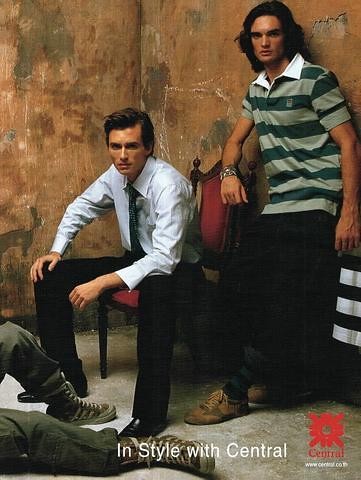In this image, a detailed setting of an old-school advertisement for a clothing brand is portrayed within what appears to be a dilapidated or abandoned building. Dominating the scene, two young men are central figures against a light warm brown wall stained with splotches of darker colors and peeling paint. On the left, a brunette man is seated in a red wooden chair, sharply dressed in a very light blue, perhaps white, long-sleeved button-up shirt paired with a dark-colored tie, black trousers, and polished black shoes. This man, with short, well-groomed hair, gazes directly at the camera. Standing beside him is another man wearing a light and darker green striped polo shirt, black trousers, and brown shoes. He has long dark hair and is slightly leaning on the back of the seated man’s chair, with green and black striped socks visible. Adding an intriguing element, the legs of a third man in green cargo pants and light brown sneakers with white laces are visible sprawled out on the floor in front of them, hinting at his presence from the left side of the frame. In the bottom part of the image, white text reads "InStyle with Central" alongside a red Central logo in the bottom right corner.